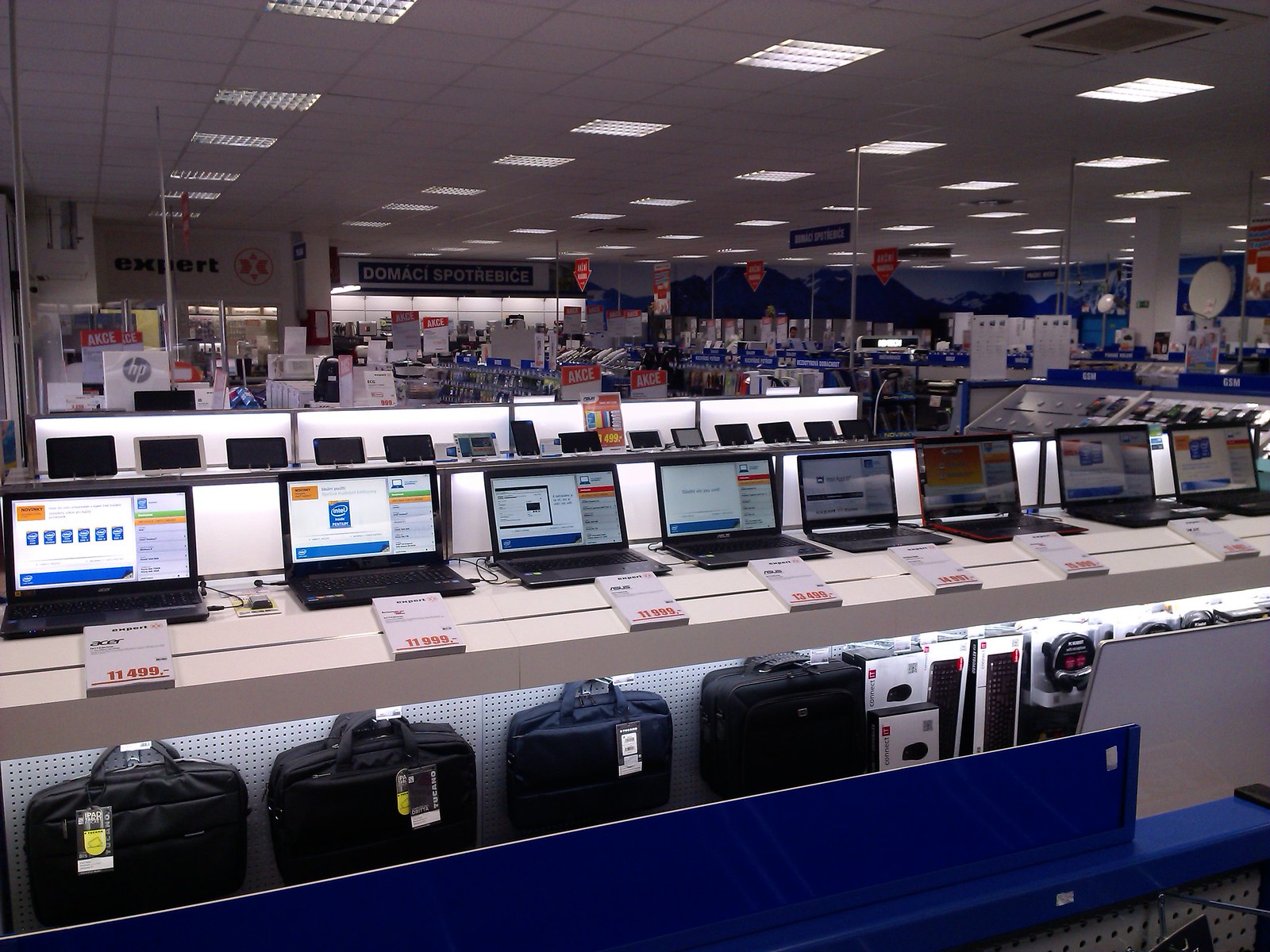This image captures the interior of a large electronics store, likely outside of America, featuring a neatly arranged display of technology products. In the forefront, a white counter showcases eight opened black laptops with active screens, aligned diagonally from the left center to the right center of the frame. Each laptop is accompanied by a white price tag with red numerals, indicating prices such as €11,499 and €11,999. Below this counter is a blue-fronted shelf holding several black laptop carrying cases alongside various computer peripherals, including keyboards, mice, and headphones. The store's aisle extends into the background, revealing rows of similar white tables brimming with electronic devices. The ceiling is a typical drop ceiling with numerous square white panels interspersed with rectangular fluorescent lights. In the distant right, other sections of the store host more electronics, discernible by a prominent, though illegible, blue sign with red letters spelling "D-O-M-A-C-I S-P-O-T-R-E-B-I-C-E." The overall ambiance indicates a bustling marketplace with an extensive inventory of technology products readily displayed for customers.